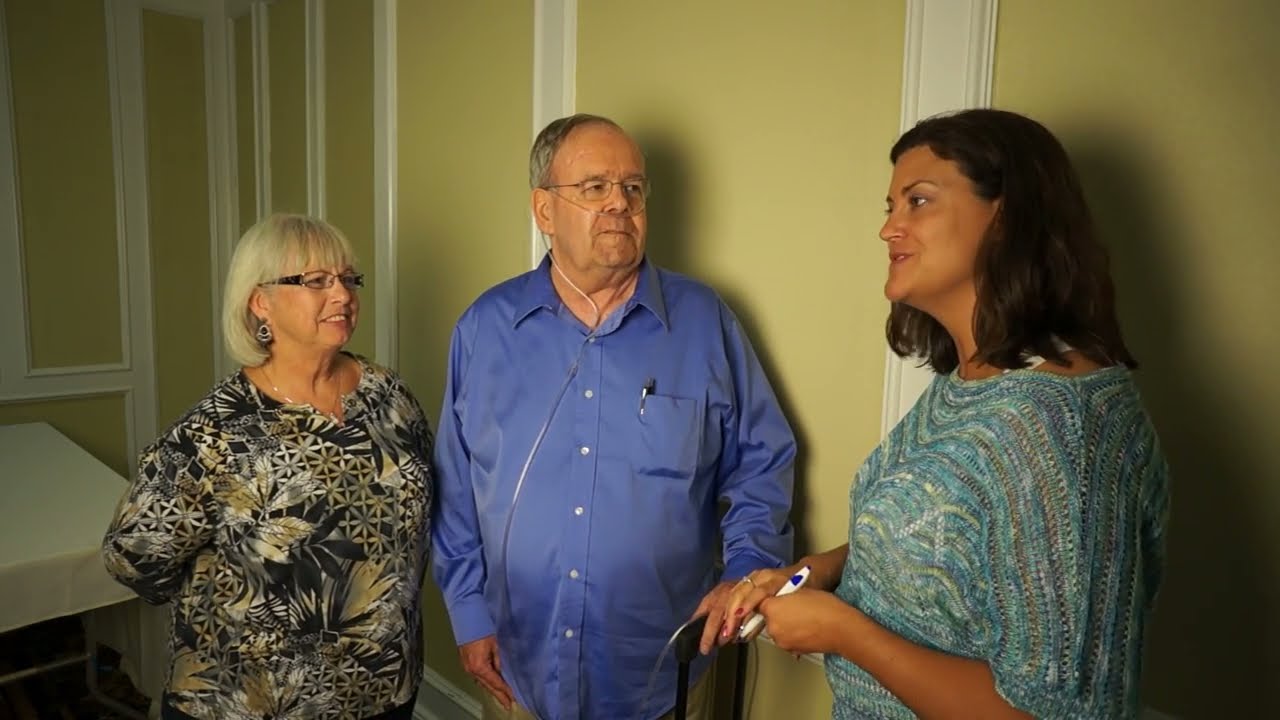In this image, three people are prominently positioned against a bright, patterned wall with a yellow and white design. Central to the scene is an elderly man, likely in his early 70s, with gray hair and a light skin complexion, wearing a blue button-down shirt with a pen in his right pocket. He has an oxygen tube connected to his nostrils, which likely runs to an unseen tank, and is holding a cane in his left hand. To his left, if you're viewing the image head-on, stands his partner, an older woman with a light complexion, blonde hair, and black-framed glasses. She is wearing a floral patterned blouse in black, gold, and white, and is listening intently. On the right, a brunette woman, presumably in her 30s or 40s, is seen in profile, engaging with the couple. She is outfitted in a teal, crocheted knit sweater, and holds a white notepad and pen in her left hand, with her arms gesturing as she speaks. Both the elderly couple are facing forward while the brunette woman is turned towards them, suggesting a conversation possibly related to medical or care instructions. In the background, behind the couple and to the far left, there is a table draped in a white cloth. The setting seems to be an indoor space, potentially a rest home or physical therapy facility.